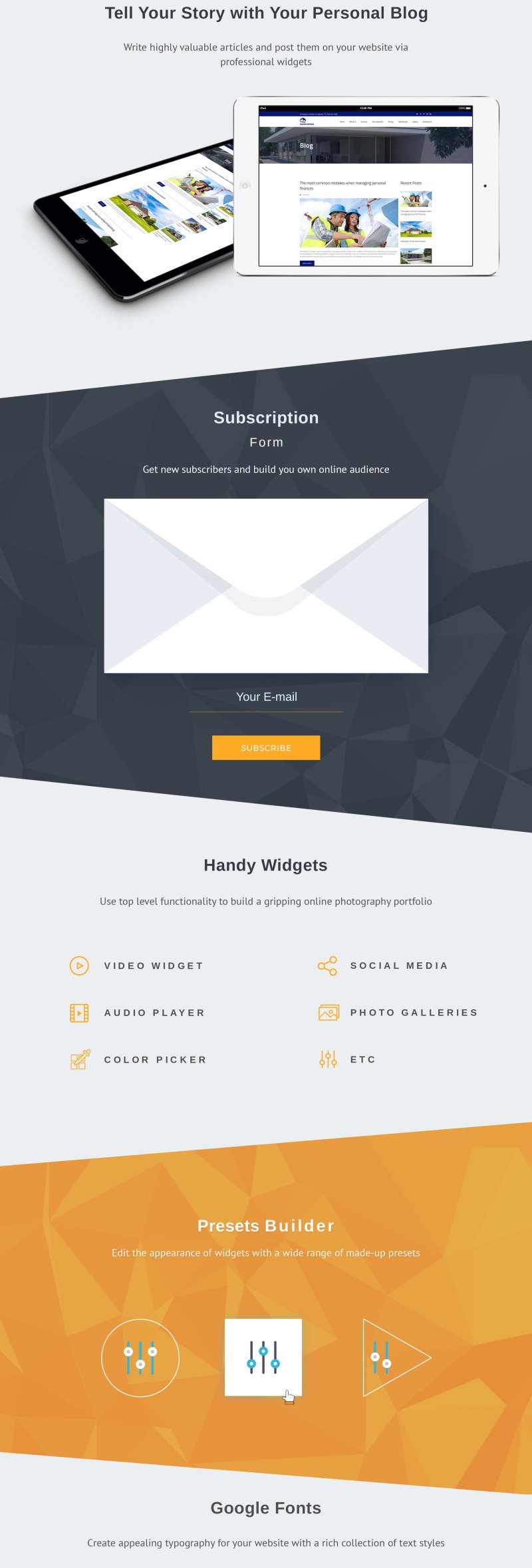A screenshot of a desktop website showcasing a sleek and comprehensive personal blog creation platform. The page features a header with the slogan "Tell Your Story with Your Personal Blog" followed by a detailed overview of tools and features. Central to the page are two high-resolution images of tablets, likely iPads, displaying vibrant blog interfaces. Further down, a subscription form invites users to "Get New Subscribers and Build Your Online Audience," highlighted by a computer-generated envelope icon, symbolizing email sign-ups. The page also boasts a variety of handy widgets, including video, audio, color picker, social media links, and photo galleries, all designed to enhance blog functionality and aesthetics. Towards the bottom, information about pre-built presets and a site builder indicate the platform's versatility and ease of use for creating a visually appealing and engaging blog.